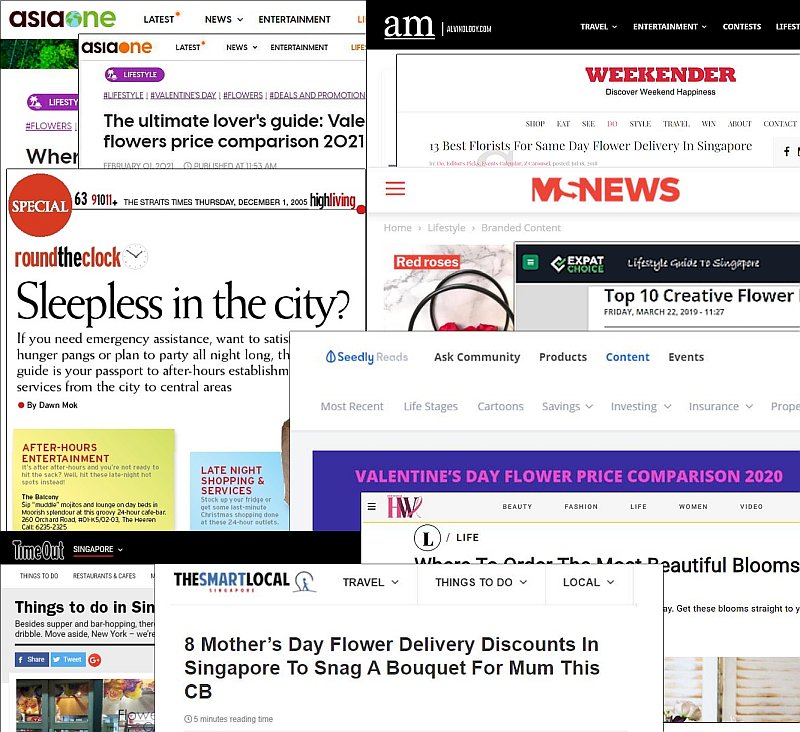An intricately chaotic screenshot displays a multitude of open windows and pop-ups, appearing as a collage of overlapping browser tabs and information. The cluttered interface highlights various content aimed at diverse users. 

Starting at the very top-left corner, the window titled "Asia 1" features a navigation bar, partially obscured by another "Asia 1" window distinguished by a slightly different logo with an orange hue and its own nav bar. 

To the right, a pop-up for "The Weekender" attracts attention with its slogan, "Discover Weekend Happiness." Moving down to the left, another promotion, "Special Round-the-Clock: Sleepless in the City," is prominently visible. Adjacent to it, on the right, is "MS News," followed on the same horizontal line by "Expat Choice: Top 10 Creative Flower."

Beneath this row, a single pop-up titled "Seedly Reads" sits on the right. At the bottom-left corner, "Time Out Singapore" lists "Things to do in Singapore," while to its right, "HW" offers guidance on "Where to order the most beautiful blooms."

Centrally positioned at the very bottom is "The Smart Local," showcasing an enticing headline: "8 Mother's Day flower delivery discounts in Singapore to snag a bouquet for mum this CB." This complex mosaic of windows forms an overwhelming yet fascinating snapshot of digital multitasking.